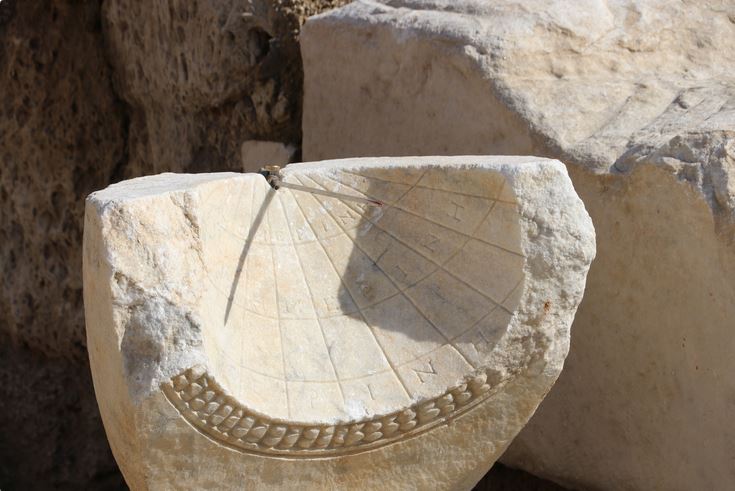This horizontal rectangular photograph captures a detailed view of various stones, likely remnants of architectural structures. Dominating the foreground is a large, cream-colored stone object that resembles an inverted bowl with a quarter-sphere shape. The interior surface of this stone is intricately carved with a grid pattern, each square housing letters such as N, I, E, and H. This finely sculpted stone, possibly part of a niche or decorative architectural element, showcases a blend of artistry and function.

To the left in the background, there is a darker, porous stone with a sandy hue interspersed with splotches of deeper brown. This piece presents a rough, natural texture with several indentations or holes, adding a raw, unrefined contrast to the smooth, carved surfaces of the foreground stone.

On the right side of the image, a large block of a similarly light-colored, cream marble stands tall. This stone, characterized by its flat surface and jagged top, appears more uniform and may have originally been a structural support or wall segment from which the foreground object might have detached. The uniformity and possible man-made aspects of this marble hint at its use in building, further suggested by the broken edges and remnants of metal reinforcements or fasteners.